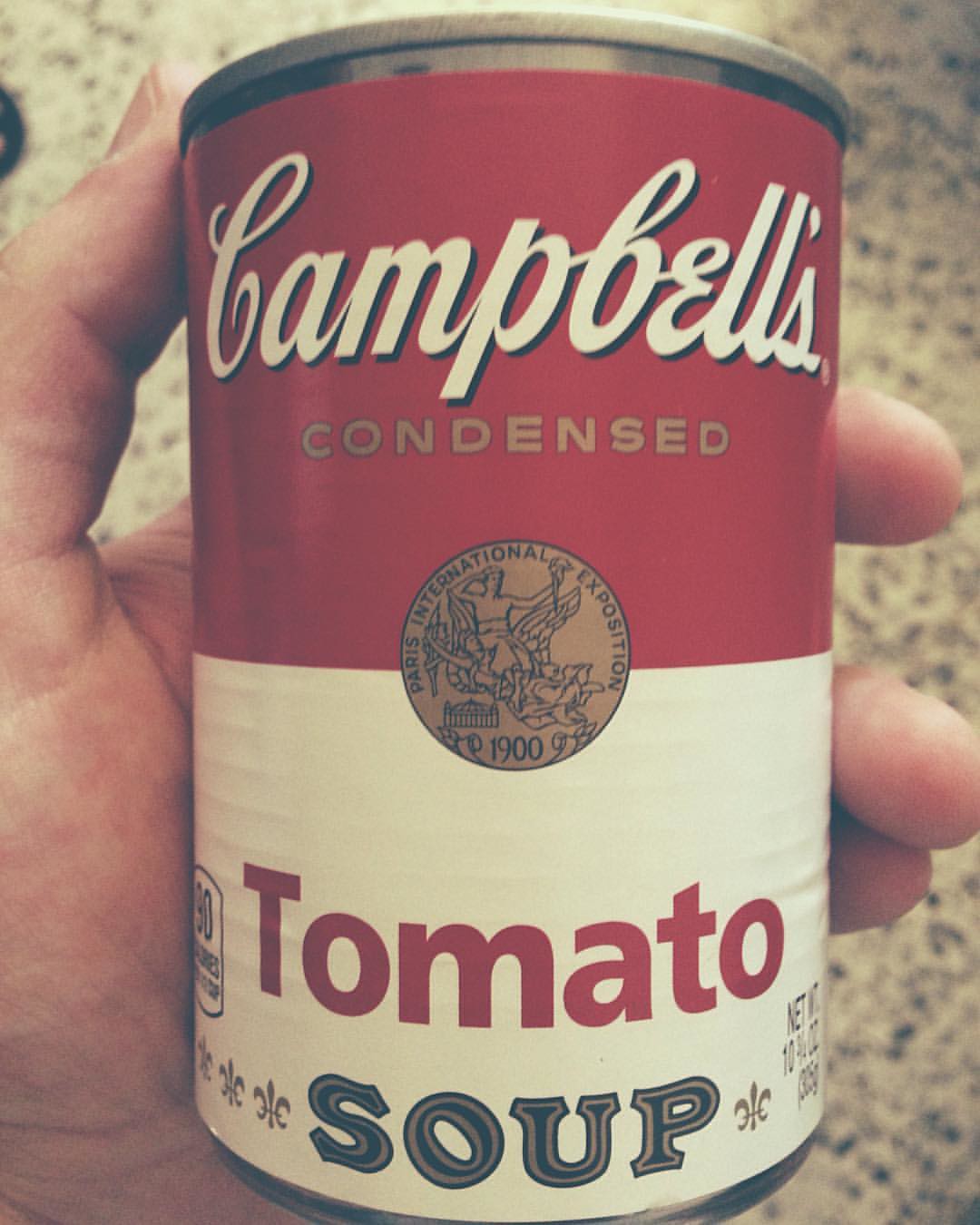A close-up photograph captures a somewhat blurry and faded image of a can of Campbell's soup. The can is held by a left hand with light skin, the thumb resting along the top rim while the fingers splay out on the right side of the can. The setting appears to be a kitchen countertop made of quartz or a similar stone, featuring a beige surface with small black speckles.

The can itself is designed with a silver-toned top and bottom, divided by a two-toned label. The upper portion of the label is a darker red, prominently displaying the word "Campbell's" in white cursive script. Below this, in smaller gold lettering, is the word "condensed." Further down on the red section, there's a gold emblem signifying the "Paris International Exposition" of 1900, though the details of the emblem's illustration are indistinct.

Transitioning to the lower section, the label shifts to white, continuing with the emblem that extends slightly from the red portion. The word "tomato" is written in bold letters, immediately followed by the word "soup" beneath it. On the left side of the white label, it likely indicates "90 calories per serving," though the text is partially obscured. On the right side, the net weight is presumably mentioned, but the specifics are unreadable.

The overall image offers a nostalgic glimpse into a classic product, framed by the everyday, textured elegance of a stone countertop.